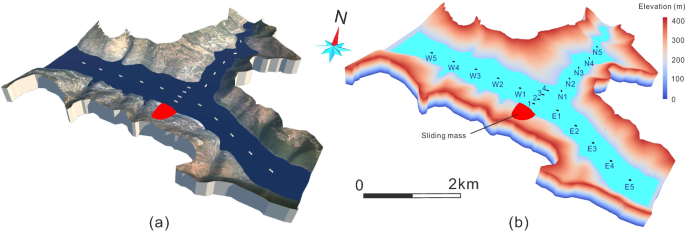The image is a detailed diagram depicting a geographical area with distinct left and right sections labeled A and B. In between the images, a scale indicating "0-2 km" with a grey notch in the middle is present. The left side, labeled A, illustrates a dark blue river or body of water with internal lines suggesting the water flow direction. The right side, labeled B, employs a gradient of bright blue, dark blue, white, and red to represent varying elevations, with a compass pointing north. Elevation indicators show that blue corresponds to zero elevation, while red signifies 400. The diagram also references a roadway, reminiscent of a coastal highway intersected by another road, with the elevation chart accurately detailing the elevation changes across the mapped area.